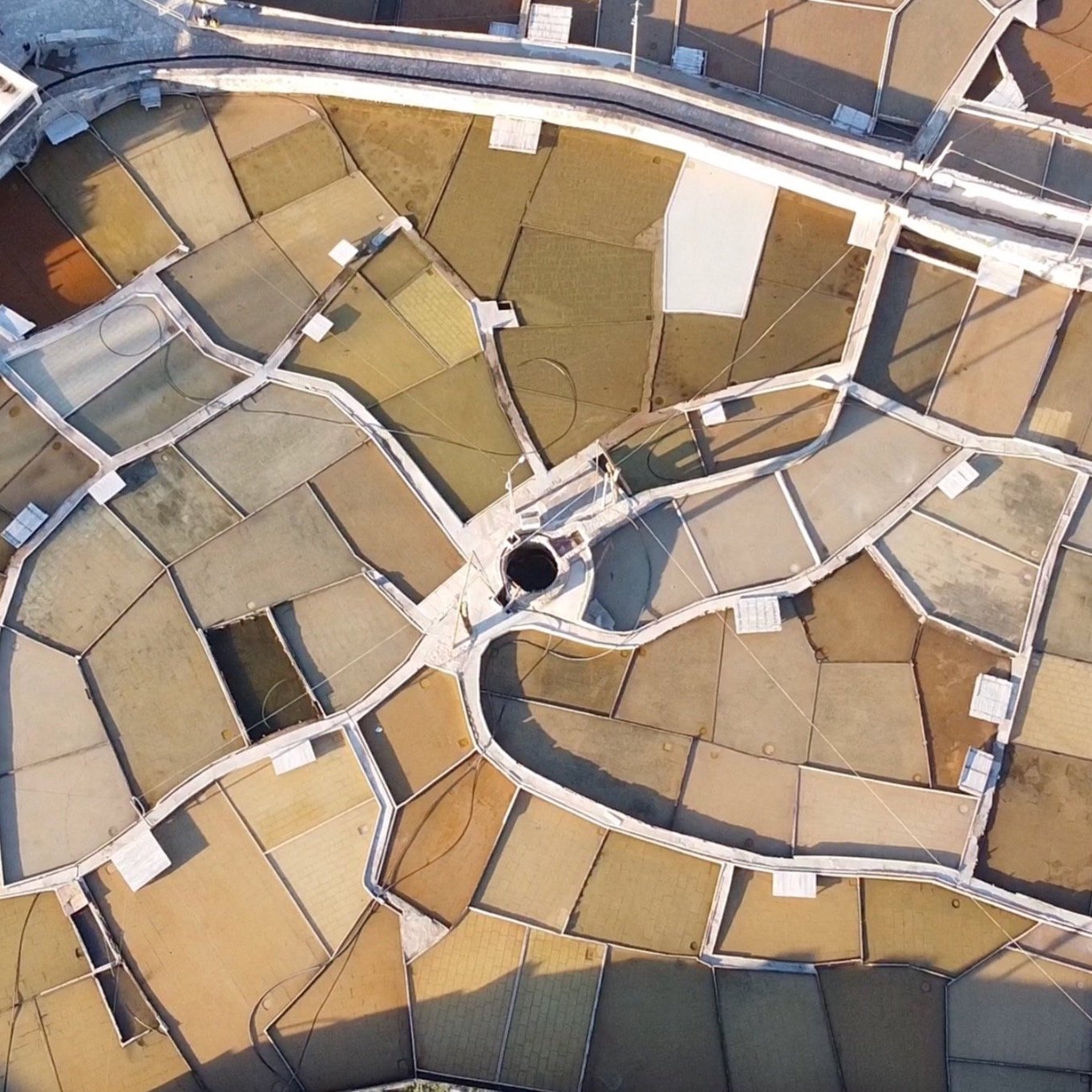This image captures an aerial view of an outdoor construction site during daylight. The scene is composed of a complex grid of interlocking sections that appear to be the roofs of buildings in various stages of completion. These sections, mostly tan, light brown, and grayish in color, are divided by white lines and barriers, creating irregular shapes—primarily squares and rectangles, but also five-sided forms with some curved walls. In the center of the image, there is a prominent round hole bordered in white, which stands out against the structured layout. Shadows cast over the area confirm the outdoor setting, emphasizing the geometric arrangement of the sections. Additionally, at the top of the image, a pathway resembling a narrow road runs from the top left to just below the top right corner, adding to the intricacy of the scene.